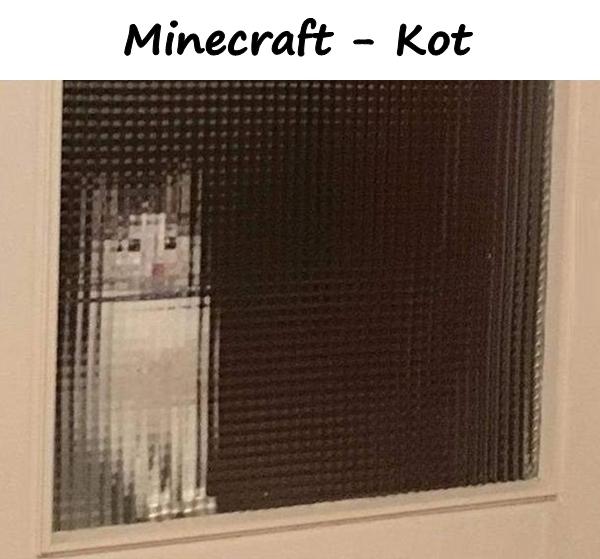The photograph captures a white cat with gray ears and black eyes, standing on its hind legs and peering through a pixelated or blurry glass window. The glass distorts the cat's figure, making it appear blocky and pixelated. The window is set in a white painted frame, and the cat's front paws rest against the windowsill at the bottom left corner of the frame. The image includes a white border at the top with black text that reads "Minecraft-KOT." The overall scene gives an impression of a cat caught in a moment, humorously resembling a character from a pixelated video game.